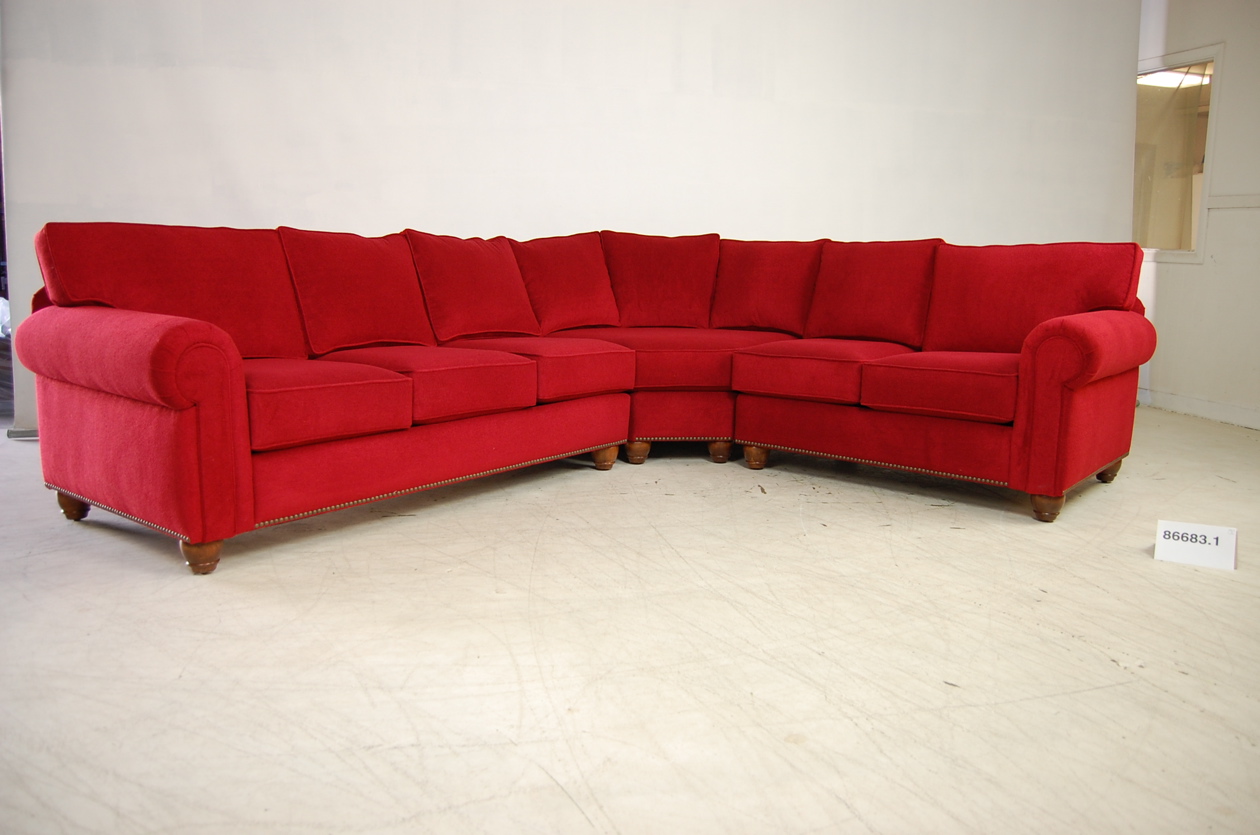The image is a realistic photograph of a large, well-lit showroom, perhaps designed to mimic a living room setting. The room features white walls and a worn, scratched tan or beige wooden floor. Central to the image is a bright red sectional couch arranged in an L-shape. The couch appears to be capable of seating six to eight people and consists of three main sections: a three-seat segment, a two-seat segment, and a corner piece that unites them. It is entirely red, including the armrests and pillows, and stands on multiple brown, rounded wooden feet—likely totaling twelve. Near the right end of the couch, there is a small white placard displaying the black number "86683.1." The background hints at a possible adjacent kitchen area, evidenced by cabinets and a fluorescent light visible on the left side of the frame.